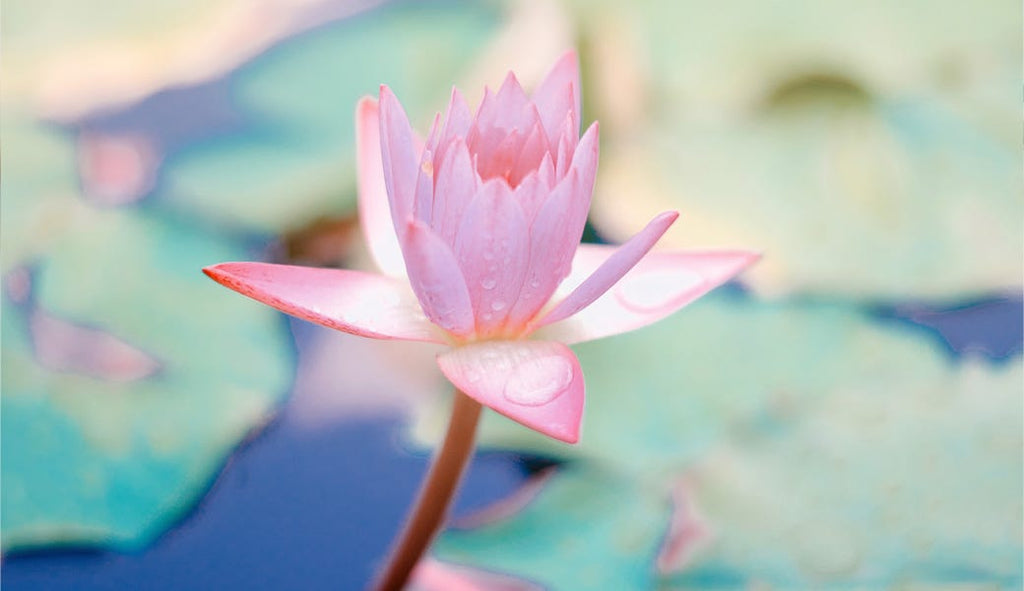This detailed photograph, taken in a landscape orientation, captures a single pink lotus flower in sharp focus against a blurred background. The flower, showcased as the central subject, has a stem exhibiting shades of brown and pink, curving gently from the bottom center toward the middle. The lotus petals, pale pink-yellow near the center and transitioning to a brighter pink at the tips, are elongated and pointed. Four of the petals are open and fanned outward, while the remaining petals are still in the process of blooming. Each petal is adorned with water droplets, with one prominent drop glistening on the petal facing the viewer. The background is artistically blurred, highlighting the plant and giving a sense of depth. Blurred lily pads in various hues—including light green, blue, tan, and cream—float atop deep blue water, enriching the color palette of the scene. This photographic representation realism captures both the beauty of the lotus and the serene aquatic environment in which it resides.